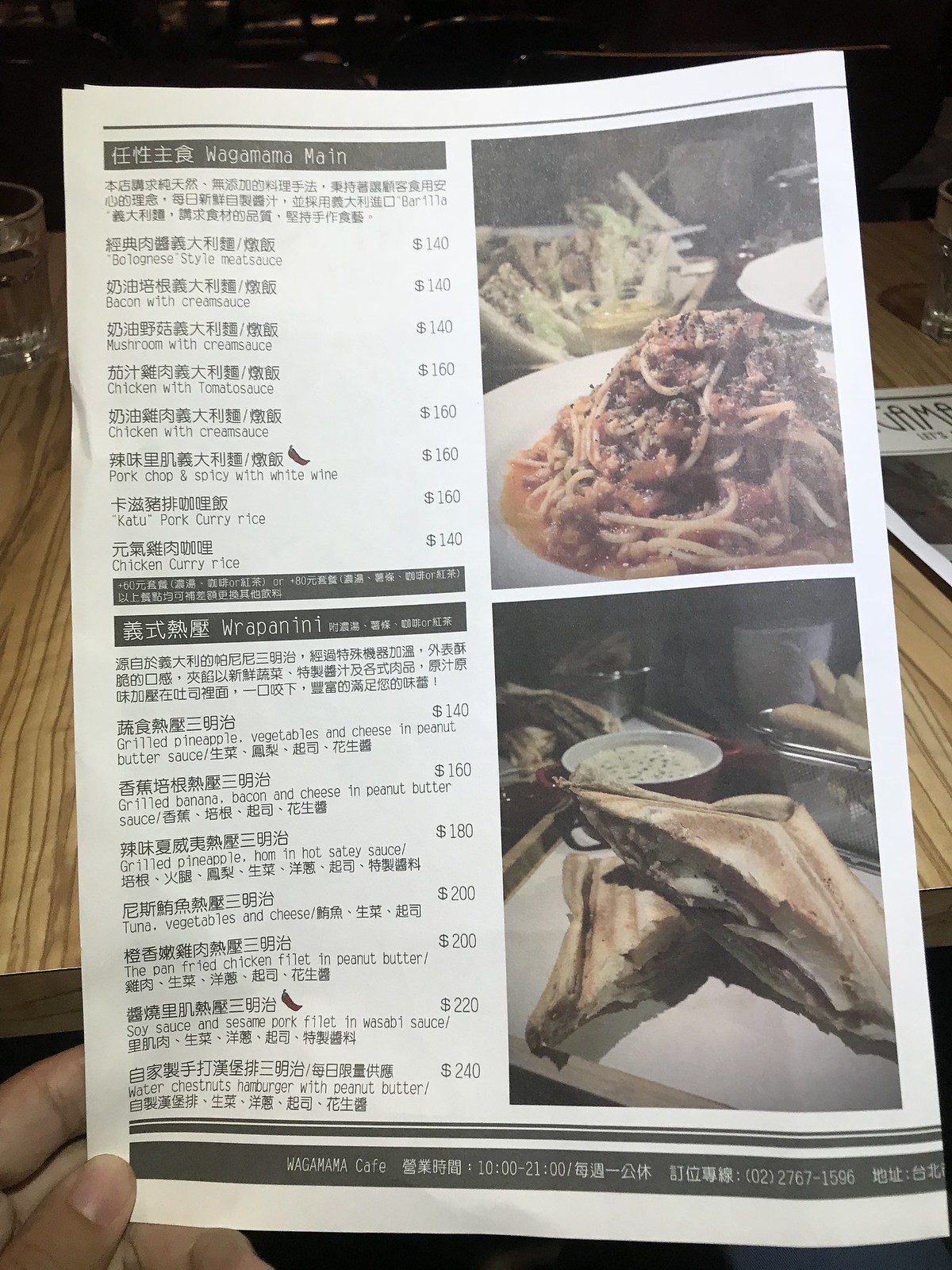The image captures a detailed view of a restaurant menu, prominently displayed at the center of the photograph. The menu, written predominantly in an Asian language with some English translations, is being held by a human hand visible at the bottom left corner of the frame. The background reveals a wooden table, adding a rustic ambiance, while on the left side of the table, there is a glass filled with water. In the dimly lit upper background, two more clear glasses and another menu are partially visible, suggesting a dining setup. The menu itself is divided into two sections on the left, bordered in black, listing various dishes. On the right side of the menu, there are two large images of food items, one at the top and one at the bottom, providing visual representations of the offerings. The English text that can be deciphered includes "Wagamama main," followed by dishes such as "chicken curry rice," "pork curry rice," "chicken with tomato sauce," "chicken with cream sauce," and "chicken fillet with peanut butter." The majority of the text, however, remains in an unfamiliar Asian script, indicating the establishment's cultural authenticity.